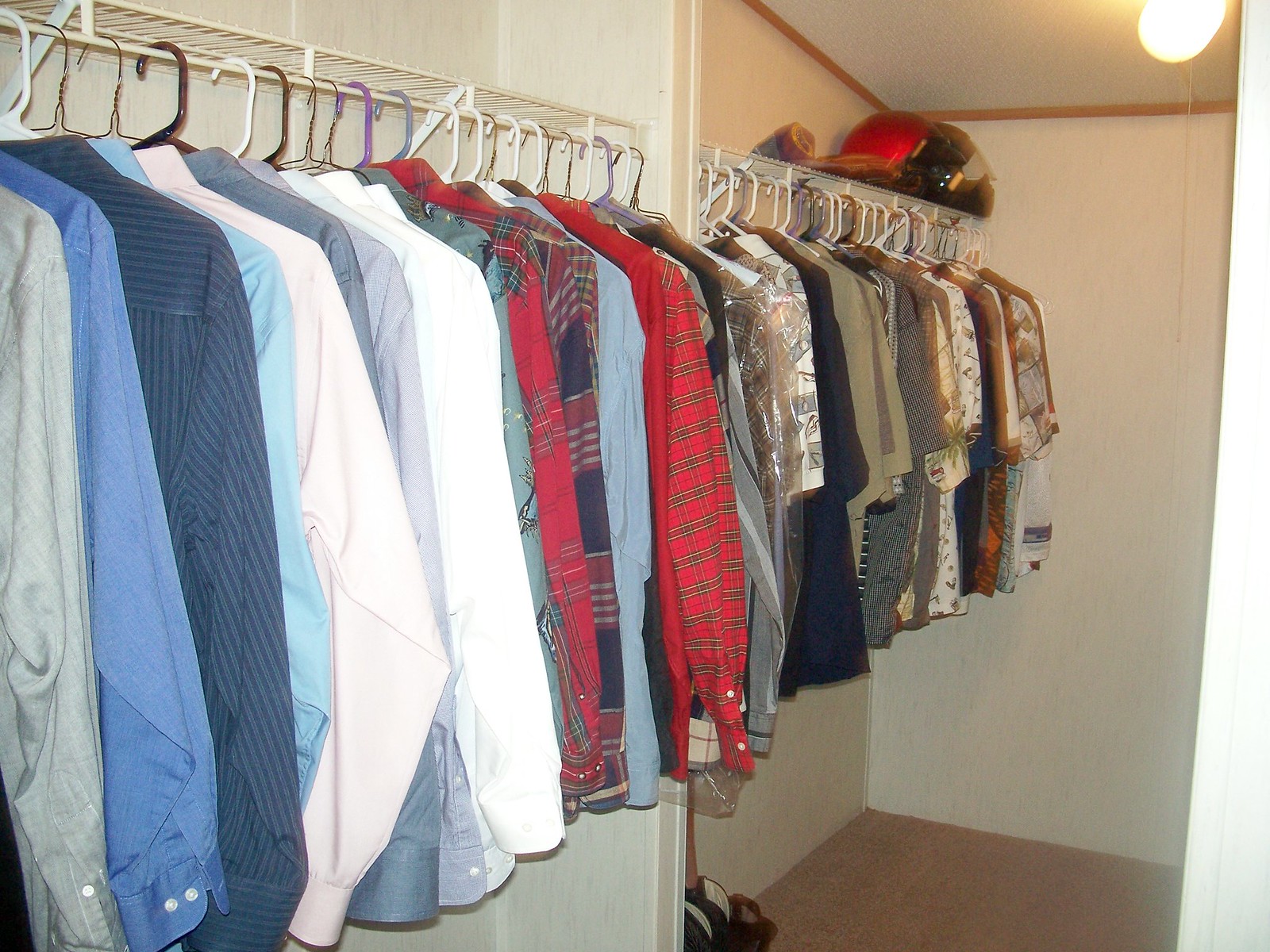This photograph offers a detailed glimpse inside a meticulously organized man's closet, viewed from a side front-facing angle. The left wall, painted white, supports a metallic bar holding an array of shirts on hangers. These shirts, mainly business casual with some white button-up options, are neatly arranged in an order from button-downs to polos, showcasing a variety of colors and designs. Above, a bright bulb illuminates the space from the right side of the ceiling. The brown floor at the bottom complements the clean walls and orderly attire. Just visible at the base are some shoes, further emphasizing the tidiness of the room.